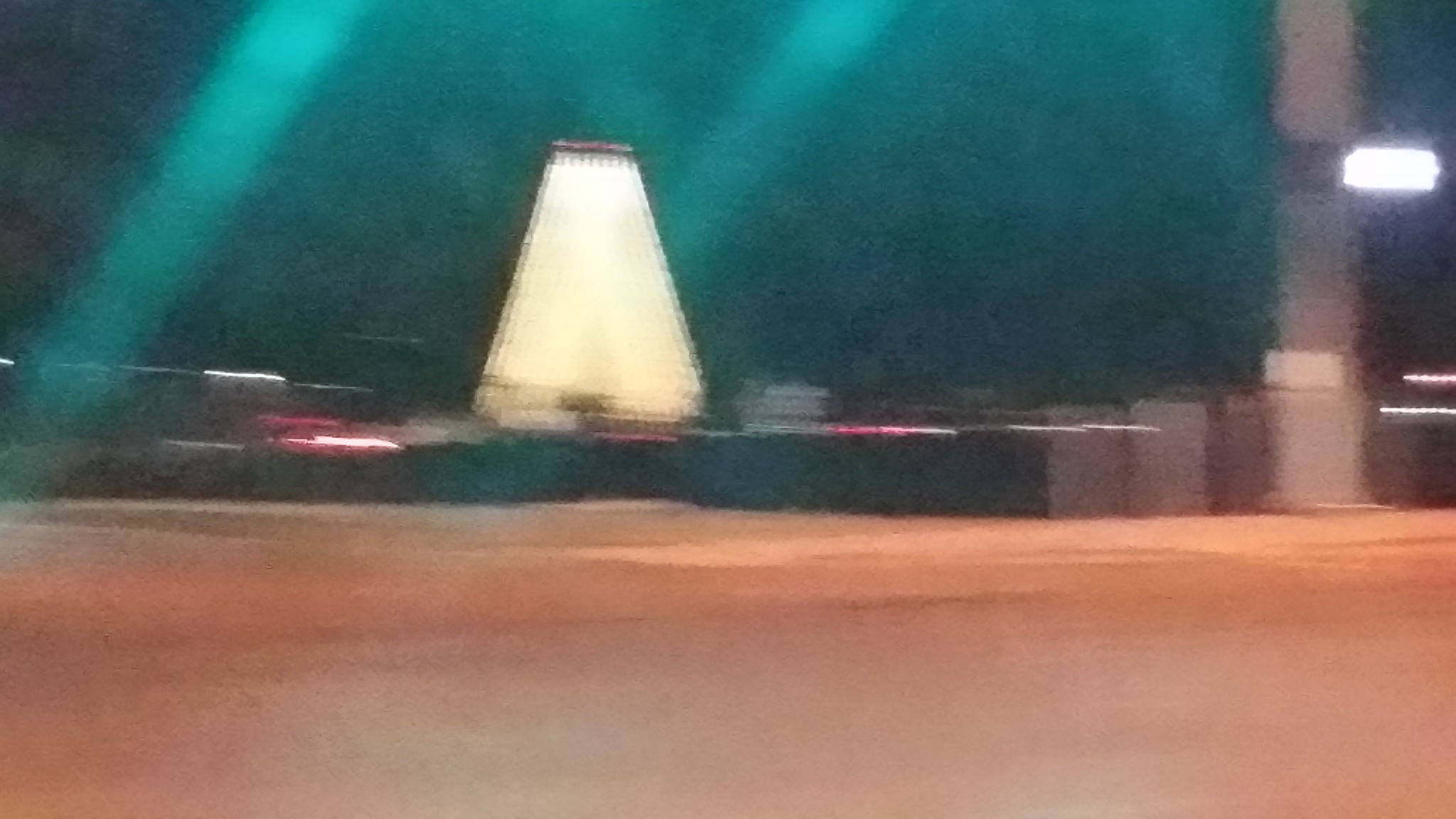A beautifully colorful, albeit very blurry and dark photograph captures a scene where details blend indistinctly. The foreground, taking up about 40% of the lower portion, showcases a rich, orangish-brown surface that could be wood or bare earth. Above this, segmented black structures stretch across, perhaps resembling a wall or indistinguishable objects stacked behind one another. Dominating the right side of the image, a gray pole extends from the bottom to the top. In the center left area, a light beams down, partially illuminating the scene. The upper half of the image remains very dark, with a few streaks and splotches of light breaking through, creating an effect akin to either a night sky with scattered lights or a dimly-lit indoor space. The photograph gives a sense of depth and mystery, with elements that are vaguely reminiscent of vehicles or containers adding to its enigma.